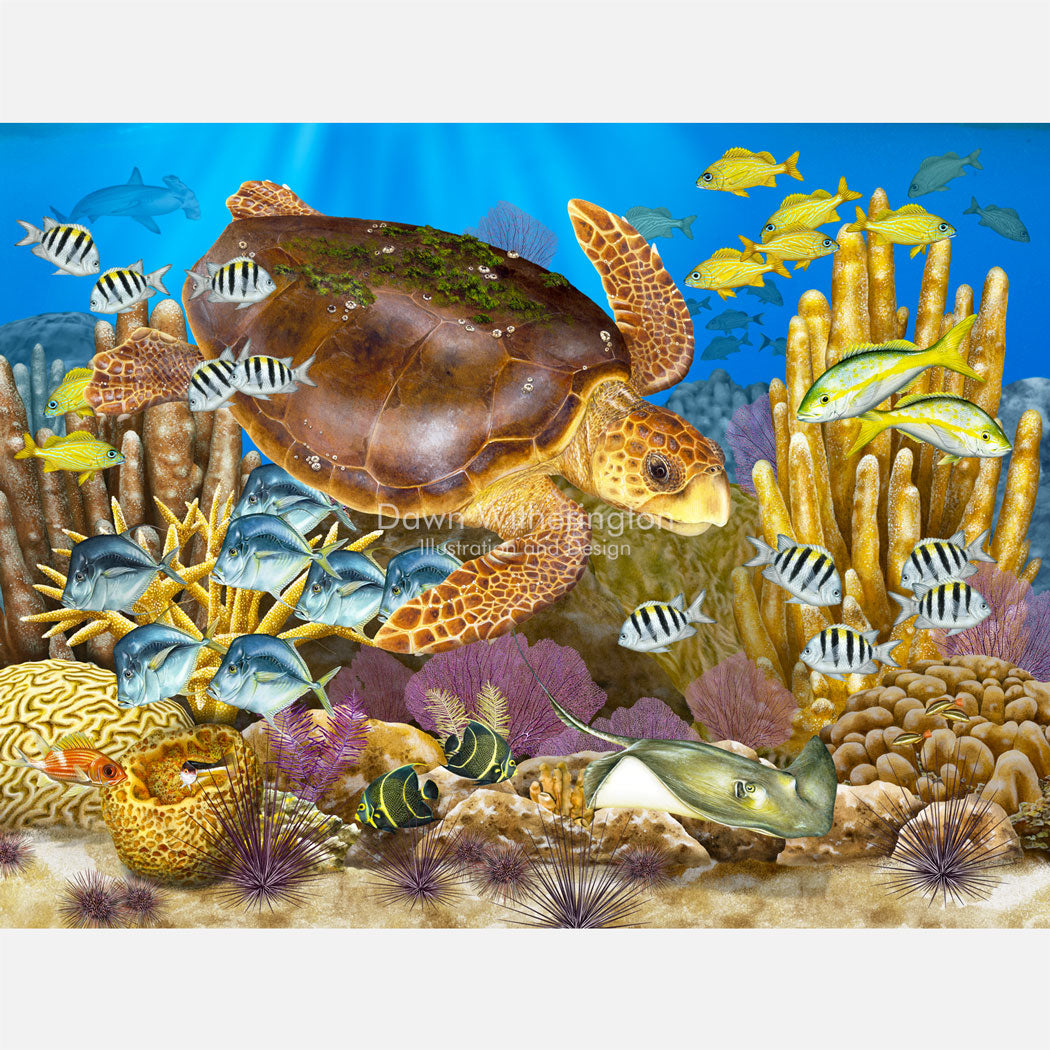In this vibrant underwater scene, the central focus is a sea turtle with a large brown shell adorned with intricate white lines and green growths, and a few white barnacle-like objects. Its body displays a rough texture, with brown and yellow patches, and it has dark eyes and a yellow beak. The turtle appears to be swimming toward the bottom right corner. The surrounding marine life includes a school of yellow fish near the top right, alongside a couple of yellow and white fish, and a pair displaying a greenish-yellow tint. To the left, there's a school of blue fish, as well as black and white striped fish that resemble zebras.

Further enriching the scene, a greyish-green stingray glides near the bottom right, accompanied by a visibly purple sea urchin. Additionally, coral reefs of various colors, such as yellow and purple, dot the sandy seafloor with its scattering of rocks and plants. A hammerhead shark can be seen in the background, adding depth to the vibrant, blue underwater setting, illuminated by sunlight filtering through the water’s surface.